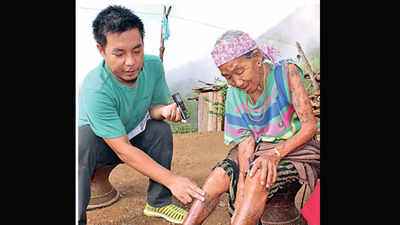In this detailed image, an elderly woman, appearing to be in her 80s with gray hair, sits on the ground. She wears a light lavender bandana and a multi-colored shirt featuring shades of green, blue, and pink. Her legs, which are brown and tan, suggest she might be in some pain or discomfort, as she is gripping one of them. Next to her, on her left, crouches a man, likely in his early 40s, who also has tan skin and short black hair. He is dressed in a light teal, short-sleeved t-shirt, dark gray pants, and lime-colored sneakers. In his left hand, he holds a black container, and he is applying what seems to be an ointment to the woman’s leg using his right hand. A white sky with a distant mountain range sets the background, while the ground beneath them is primarily dirt, hinting at a field setting. The overall scene exudes a sense of care and concern as the man attentively tends to the elderly woman's leg.